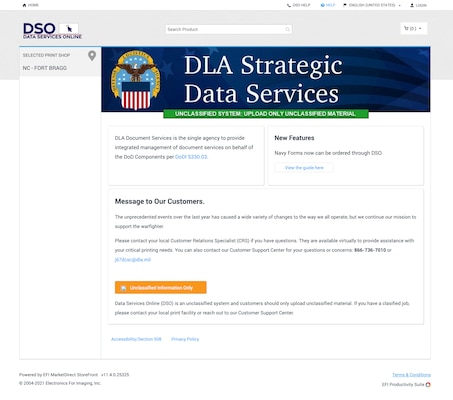The top left corner of the image features a blue header with the text "DSO Data Services Online" accompanied by a small white icon that includes a black, mouse-like symbol. Positioned at the top left is a home icon. The resolution of the page is not the best, thereby making it somewhat challenging to discern all the details clearly.

On the top right, the image displays options like "Help," "English," and "Login." Directly below these options is a white search bar with the prompt "Search Product." Underneath the search bar, a prominent blue banner reads "DLA Strategic Data Services" in white text. To the left of this banner is a logo depicting an eagle, the U.S. flag beneath it, and a background featuring a yellow ribbon with some text inscribed on it.

Beneath the blue banner, there's a green bar with black text stating, "Unclassified System – Upload Only Unclassified Material." Following this, the text in black and green specifies, "DLA Document Services is a single agency providing integrated management of document services on behalf of the D.O.D. (Department of Defense) components." Due to resolution issues, some words are difficult to decipher. 

Additional elements include a note about "New Features," stating that "Navy forms can now be ordered through D.S.O." along with a "View the Guide Here" button. Subsequently, a section titled "Message to Our Customers" is followed by an orange button and further text below it, which remains indistinct due to image clarity.